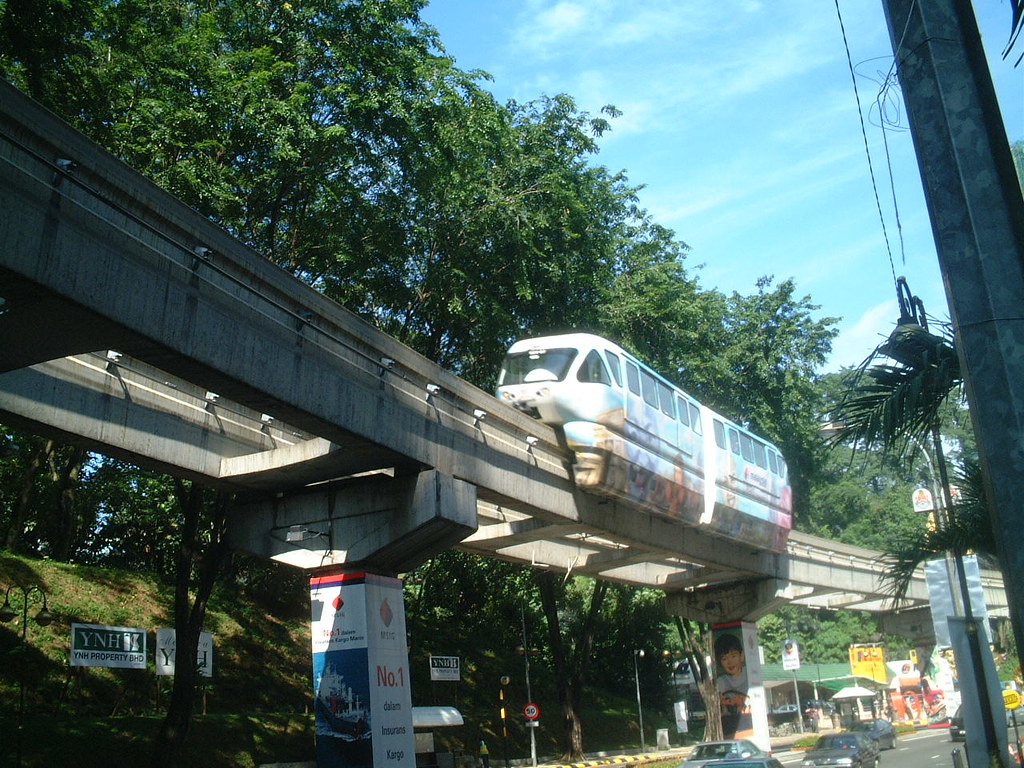The image captures a white monorail adorned with indistinct art on its left side, gliding along an elevated concrete track supported by black stanchions. The monorail features numerous windows, emphasizing its sleek and modern design. Situated within a lush, green area, the background showcases tall trees and a bright blue sky adorned with wispy clouds, indicating a clear day. Below the monorail and the track, the ground slopes down to a hilly, grassy area leading to a busy street, where a parking lot with several parked cars and moving vehicles can be seen. Notably, there are signs underneath the monorail, including an advertisement for "YNH Properties." The scene is framed by a black metal bar extending upward to the right, adding an industrial element to the otherwise serene environment.